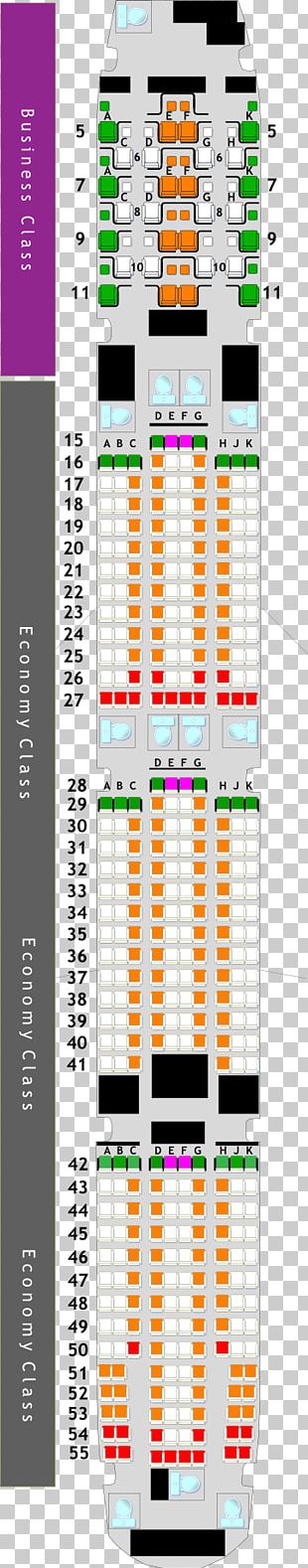This image shows an edited photo of an airplane cabin removed from its original background and placed against a background of white and gray squares. The cabin seating is organized with numbered rows and lettered categories. Along the left side of the image, there is a vertical panel detailing the seating classes. At the top left, "Business Class" is labeled, and to the right, the front of the plane is visible.

The cabin seats are colored according to their arrangement: green for the seats on the left and right sides, and orange for those in the center. Specifically, the first seats in the top left and right are numbered 5, and the second seats on both sides are numbered 7. The central seats are labeled with letters B and G and do not have numerical labels.

The first large section of the aircraft includes rows labeled A, B, C, D, E, F, G, H, J, and K, numbered from 15 to 27. The next section also follows this label pattern, with rows numbered from 28 to 41. The final section extends from rows 42 to 55. While most seats are orange, the back rows of the first and last sections are distinctly red.